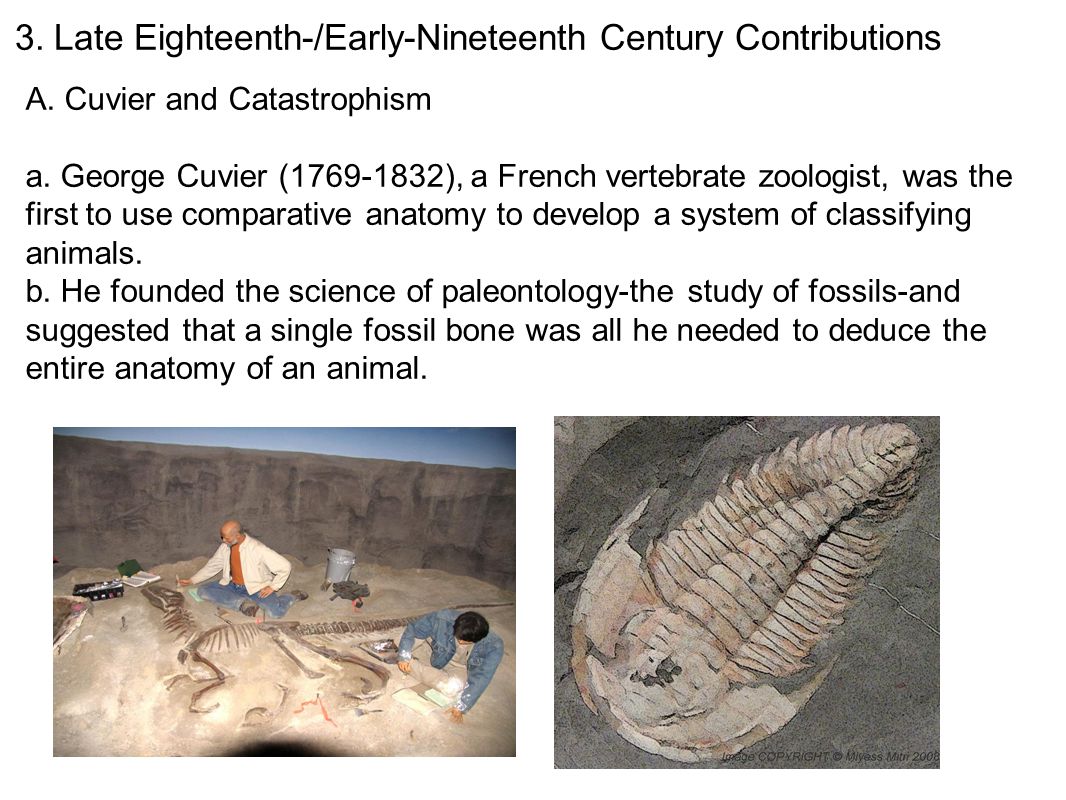The image appears to be extracted from a paleontology or zoology reference text, possibly a dictionary, encyclopedia, or textbook section on historical contributions. The white background features text at the top and two images at the bottom. The text is left-aligned and begins with the title: "3. Late 18th - Early 19th Century Contributions," followed by the subheading "A. Cuvier and Catastrophism." Below this, in smaller text, is "a) Georges Cuvier (1769-1832), a French vertebrate zoologist, was the first to use comparative anatomy to develop a system of classifying animals." This is followed by "b) He founded the science of paleontology—the study of fossils—and suggested that a single fossil bone was all he needed to deduce the entire anatomy of an animal."

Centered below the text are two images. The left image is rectangular and depicts two men: the first man, leaning down, examines what appears to be the spine of a fossil, while the second man in a denim jacket with black hair looks at some papers. The right image is square, showcasing a light gray trilobite fossil with horizontal grooves against a rocky background. The descriptive accompanying text and imagery highlight the impact of Georges Cuvier's contributions to zoology and paleontology.